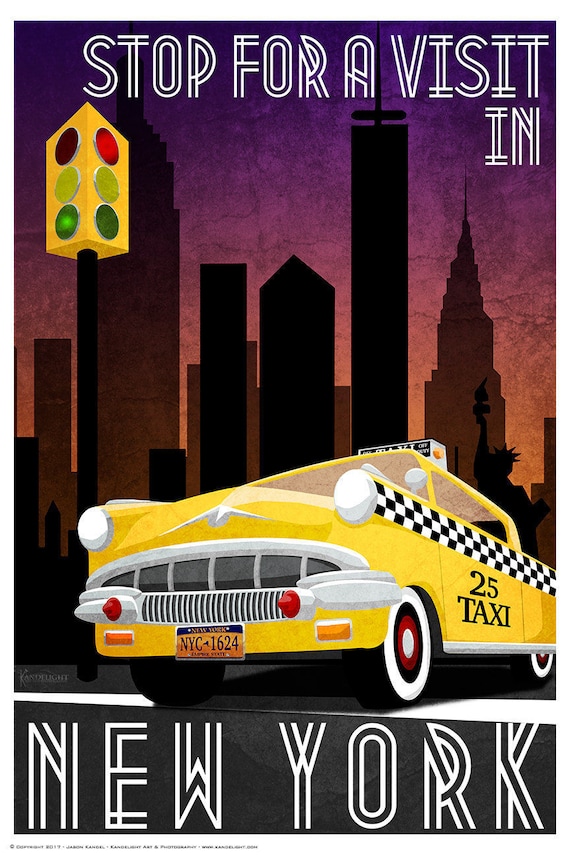The image is a detailed, computer-rendered piece of Art Deco-inspired artwork. It features a yellow taxi cab with a black and white checkerboard stripe on its side, labeled "Point 5 Taxi" in black text on the driver's door. The taxi, equipped with large chrome grilles, white wall tires, and an orange license plate marked "NYC 1624," stands prominently in the foreground, facing towards the camera and slightly to the left. The background showcases a stunning New York City skyline at dusk, with the sky featuring hues of purple and orange. Key landmarks like the silhouette of the Statue of Liberty on the right and the Empire State Building slightly to the left are visible amidst tall skyscrapers. A yellow traffic light, attached to a black pole, stands to the left of the taxi. At the top, in bold double-lined white text, it reads "Stop for a Visit Inn," while at the bottom, it is simply labeled "New York." This captivating image serves as an evocative advertisement for New York City, inviting viewers to "Stop for a Visit in New York."